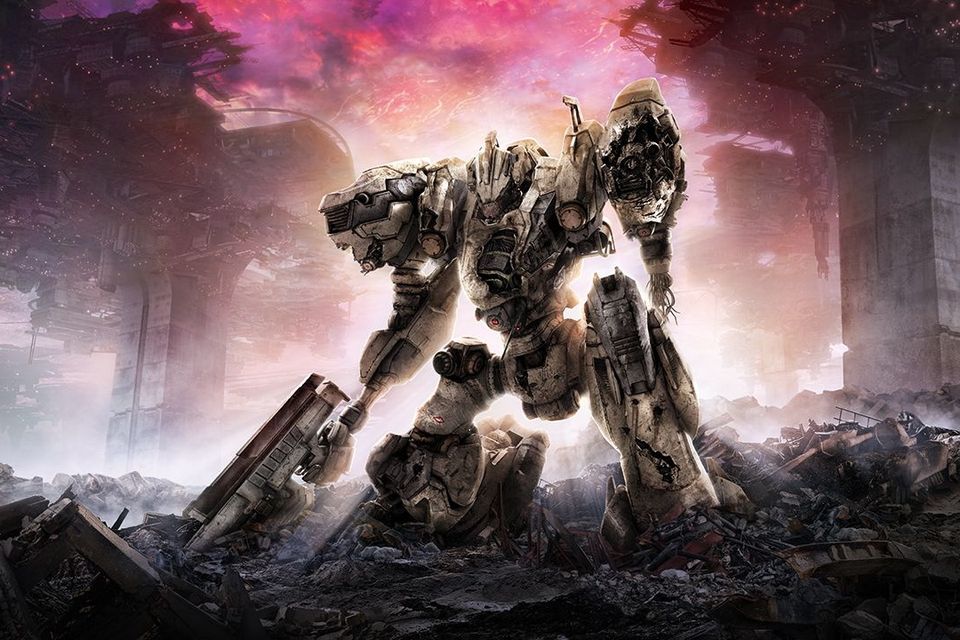The image depicts a large, transformer-like robot set against the striking backdrop of a dystopian world. The sky is awash in dramatic hues of bright white, reddish-pink, and purples, suggesting explosions or powerful light sources behind the robot. The city itself is in ruins, with collapsed bridges, torn-apart roads, and debris scattered everywhere. The robot, primarily white with touches of gray and brown, stands out in the scene. It is large, with big legs and arms, although its left arm is missing halfway, exposing wires and damage that imply recent combat. In its right hand, it holds a substantial weapon, and despite its battered appearance, it seems to be either kneeling or trudging through the rubble. The overall atmosphere of the image is dark and dystopian, highlighting a post-apocalyptic battle scene devoid of any other life forms, whether human or mechanical.